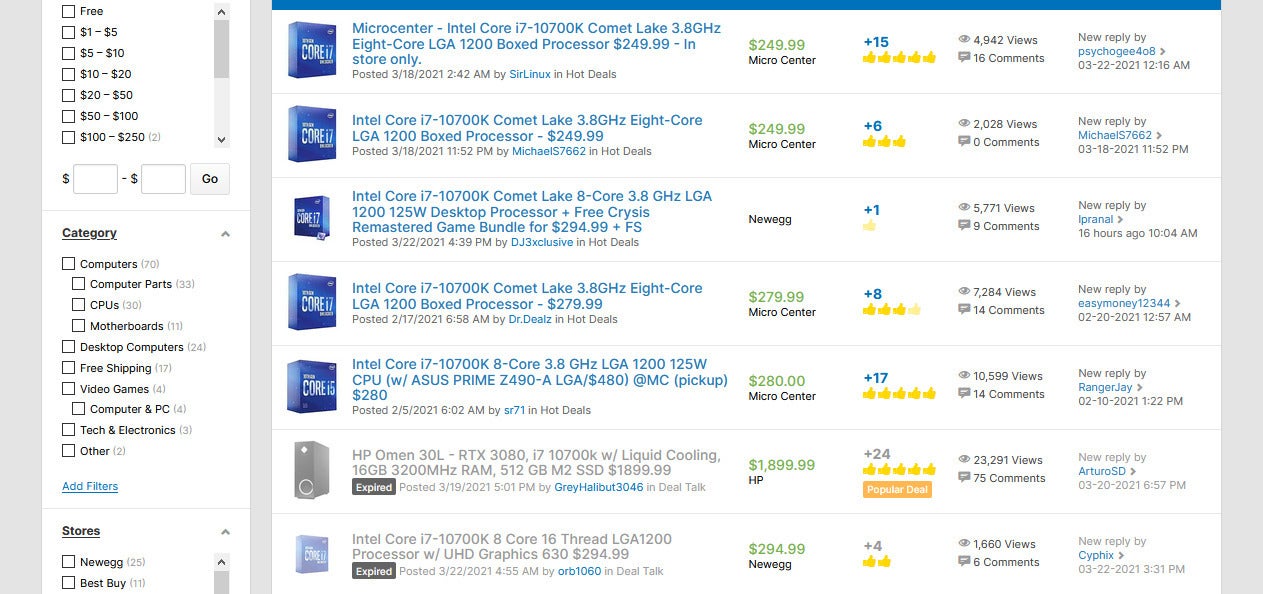This image showcases a search results page from an unidentified website, as the top part is cut off. On the left-hand side, there is a black sidebar set against a white background with gray margins, featuring various search categories to refine search results. The main section on the right lists multiple processors. Each item in the list includes details: the price is displayed immediately to the right of the processor name, followed by the rating. Next to the rating is the number of views for each processor, and lastly, on the far right, is the count of new replies.